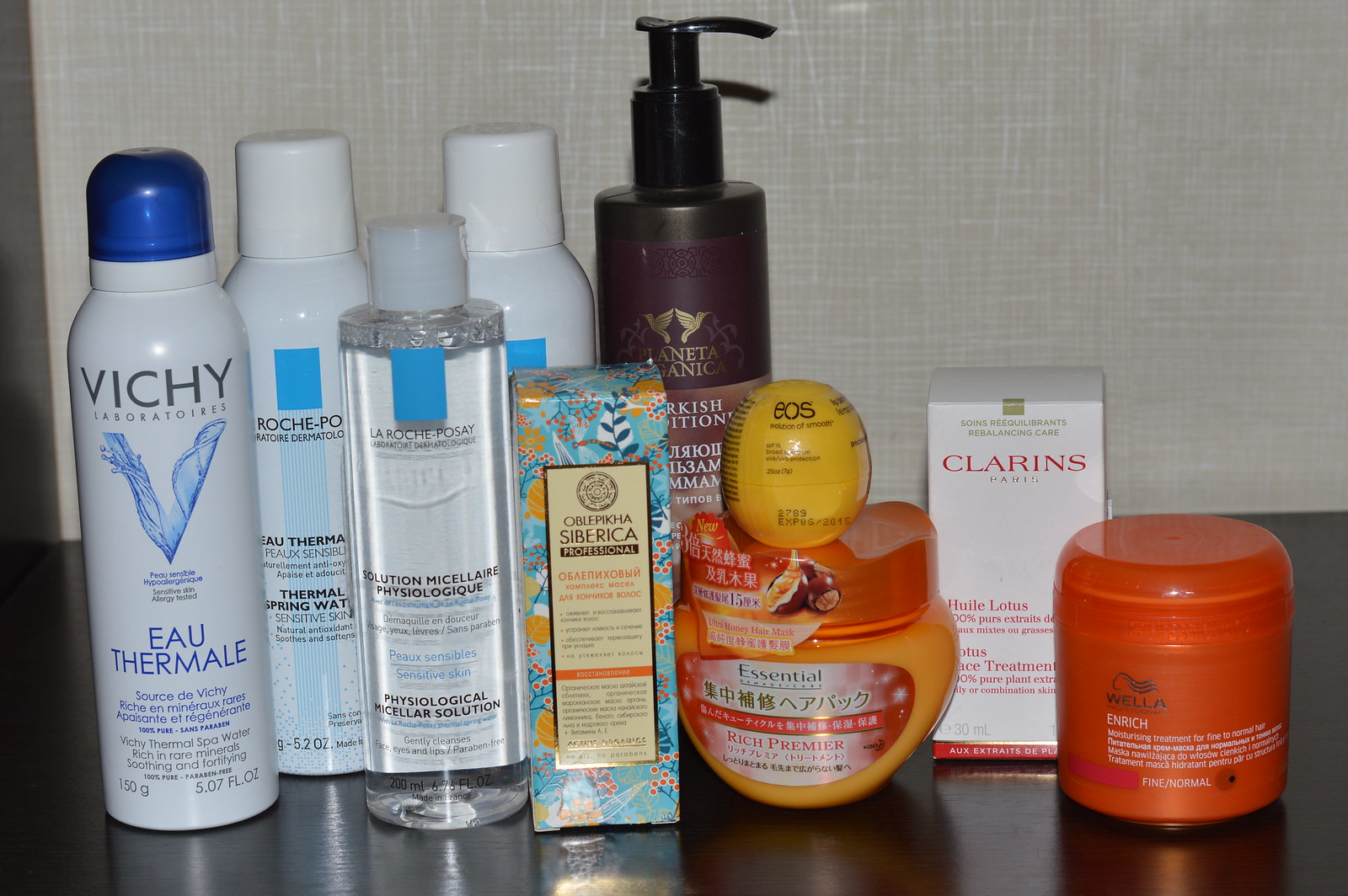An array of nine beauty products arranged neatly on a polished brown wood table against a backdrop of beige crosshatched wallpaper. From left to right, the collection includes Vichy Laboratories Eau Thermale and La Roche-Posay Thermal Spring Water, followed by La Roche-Posay Micellar Water. Next, a similar container, likely another La Roche-Posay Thermal Spring Water, though the label isn't visible. Also featured is a floral box labeled in a foreign language, presumably a product from Syberica. The lineup continues with a tall brown bottle with a spout, a squat orange jar labeled "Rich Premier" cream, and an Eos lip balm. Lastly, there's a Clarins Lotus Oil box and a Wella Enrich Treatment jar, completing this diverse selection of beauty essentials.